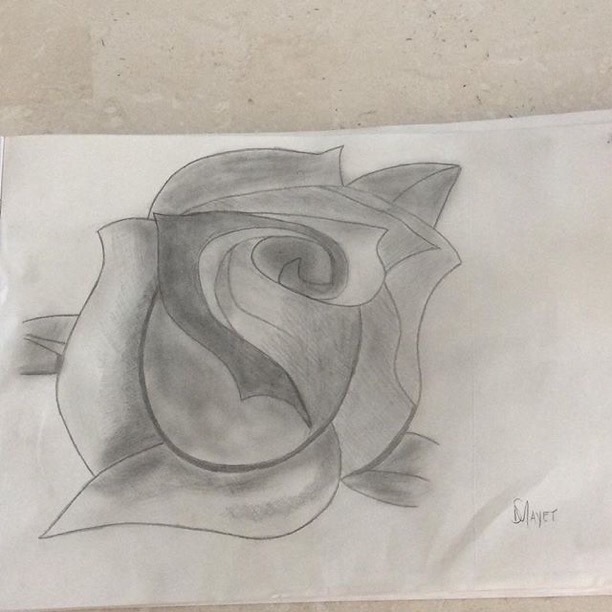This detailed pencil sketch of a rose is drawn on a small, rectangular, white sheet of paper that resembles a napkin. The sketch artist, possibly named D. Mayer, has signed the work in the lower right corner. The rose is depicted without a stem, focusing exclusively on the blossom, which is about halfway between the bud stage and full bloom. The petals are meticulously shaded to create a textured and three-dimensional appearance, with swirls and darker pencil strokes adding a touch of stylization. This attention to detail gives the rose a lifelike quality, despite its simplistic elegance. Surrounding the blossom, there are two leaves—one positioned at the upper right and the other at the middle left. The paper itself appears to have slight wrinkles or shadows, enhancing the sketch's authenticity. The background reveals a tiled surface, suggesting the image might have been taken in a classroom or similar setting.